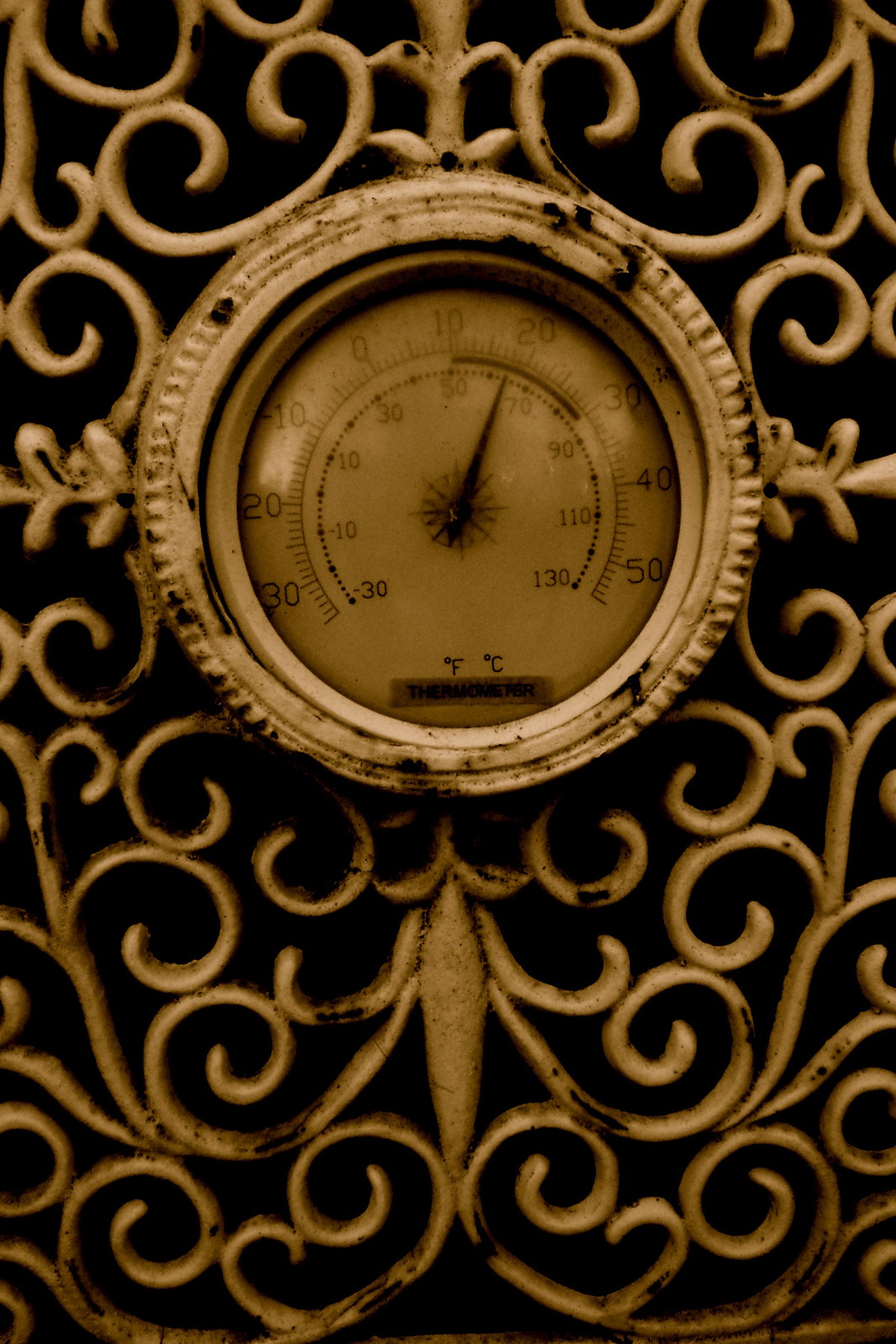The image features a detailed clock timer crafted from a white ceramic or metallic material. At the center, a thick white ceramic circle houses the timer's face. The face is marked with numbers in increments of 10, starting with 0 at the top left, followed by 10, 20, 30, 40, and 50 arranged clockwise. Inside this primary circle, a semi-circle can be observed displaying larger numbers – 50, 70, 90, 110, and 130 – in a clockwise sequence around its perimeter. Surrounding the timer face is an ornate design of intricate filigree metal shapes, adding an element of artistic elegance to the functional device, akin to an elaborate clock face.